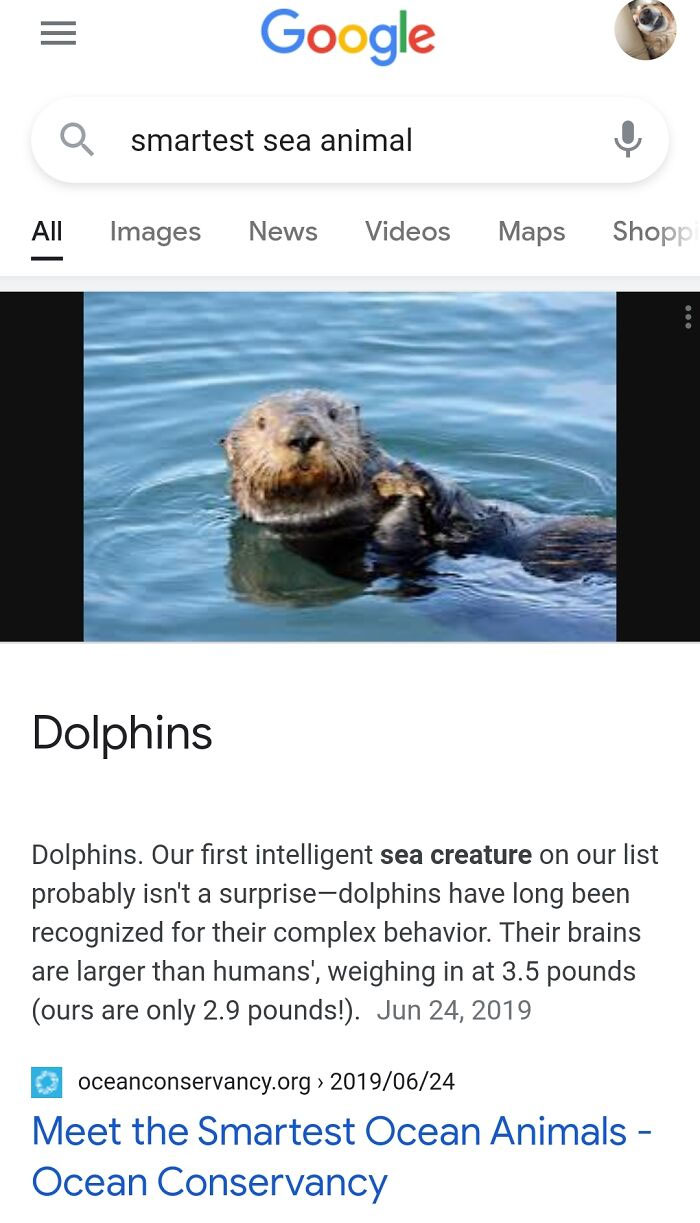**Detailed Caption:**

This image is a mobile phone screenshot capturing a Google search result for the query "smartest sea animal." At the top left corner of the screenshot, three horizontal bars serve as a menu selection option, while the center displays the iconic multicolored Google logo in blue, red, orange, and green letters. On the upper right corner is the user’s avatar, which features a cute dog with its head tilted to the side.

Below the logo and avatar is the search box with rounded corners. The left side of the box holds a magnifying glass icon, the center contains the text "smartest sea animal" in all lowercase letters, and the right side features a microphone icon. Beneath the search box are the various Google search options: "All," "Images," "News," "Videos," "Maps," and "Shop," with "All" being currently selected and highlighted in black text, while the other options appear in light gray.

The main search result in the center showcases an image that appears to be of a sea otter, although the search query is about dolphins. The sea otter in the image is facing the camera with its body submerged in deep water; the photo has black edges on the left and right sides. Below the image is the text "dolphins" in bold, and the subtext describes dolphins as the "first intelligent sea creature." It emphasizes, "probably isn’t a surprise, dolphins have long been recognized for their complex behavior. Their brains are larger than humans, weighing in at 3.5 pounds. Ours are only 2.9 pounds." 

The source of the information is noted as "OceanConservancy.org," dated June 24, 2019, with the URL title "Meet the Smartest Ocean Animals - Ocean Conservancy." To the left of the URL is a small blue square icon featuring a white wreath circle. The text from the search result is dated June 24, 2019, as seen in light gray beneath the descriptive content.